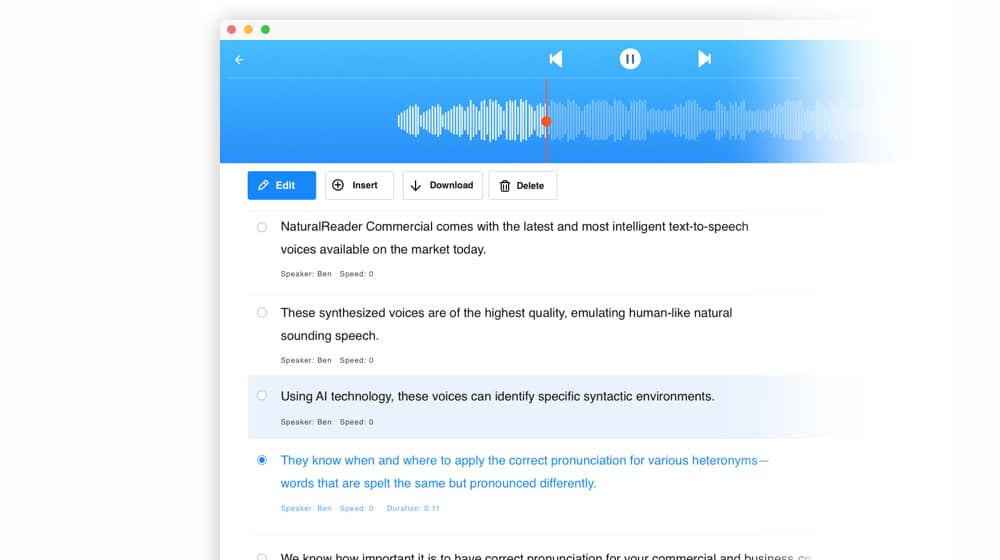The image depicts a web page interface for a blue sound box designed for audio playback. At the center of the interface is a prominent blue sound box with a clearly marked button for activating audio, which could be a recording of someone speaking or music. Below the sound box, there is a row of four buttons, each featuring distinct icons labeled "Edit," "Insert," "Download," and "Delete" from left to right.

Further down, multiple text-to-speech options are listed. Each option is introduced with "Speaker, Ben, speed zero" and elaborates on advanced features. The first option highlights the cutting-edge, human-like quality of the text-to-speech voices, noted for their commercial-grade naturalness. The second option emphasizes the sophisticated AI technology that these voices use to accurately navigate complex syntactic environments. This option is visibly highlighted in blue. The third option details the adaptive pronunciation capabilities of the voices, especially useful for heteronyms—words that share the same spelling but have different pronunciations. This choice is marked as active with a blue button, indicating its selection. The duration of this specific choice is mentioned as 11 seconds.